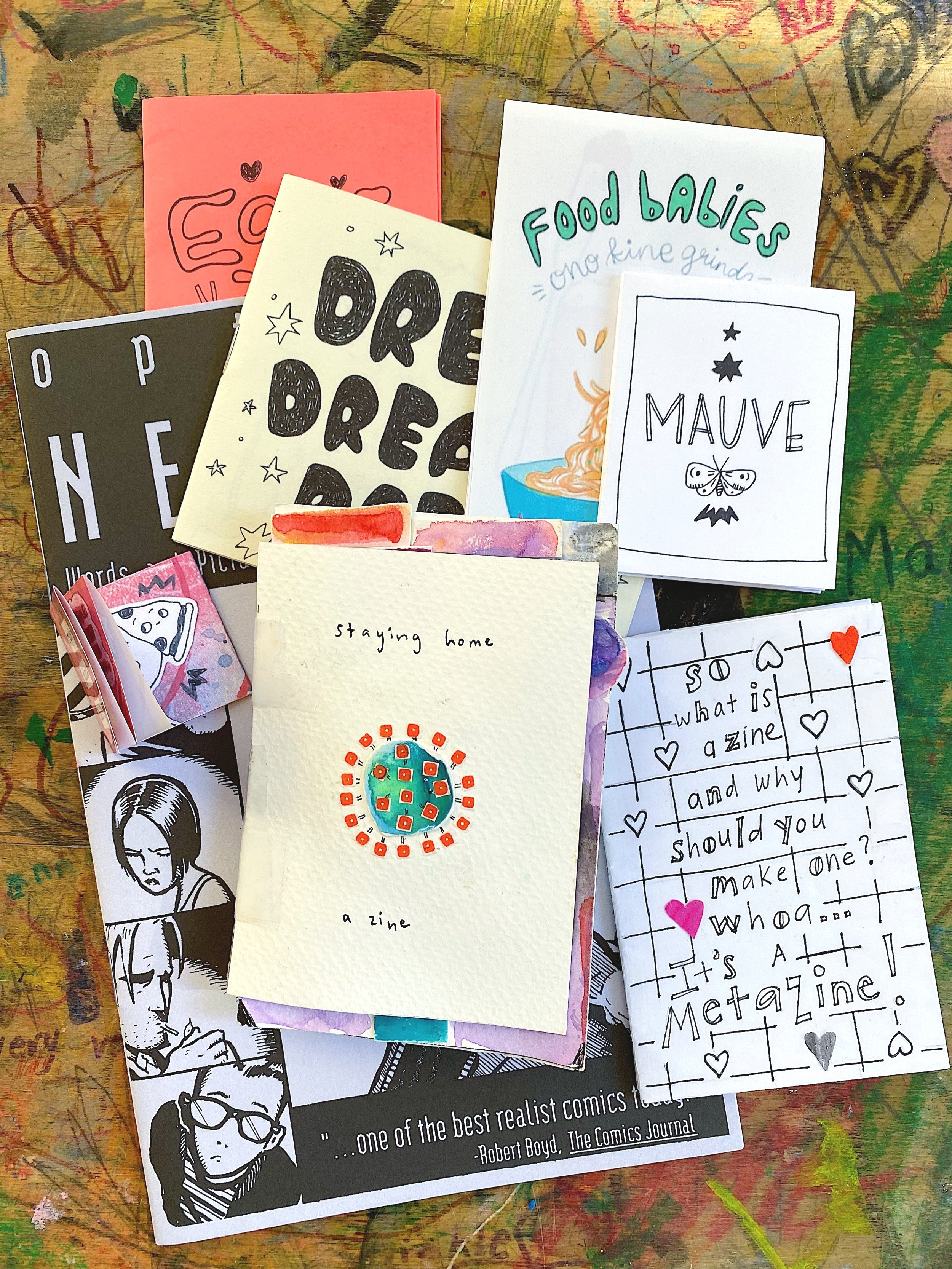The photograph showcases a vibrant collection of handmade zines, postcards, and paper crafts, all intricately layered and partially overlapping each other on a vividly illustrated poster board. Dominating the topmost visible items is a zine titled "Food Babies," adorned with a child's drawing. Nearby, another zine named "Mauve" appears with a picture of a moth featuring three black stars. There's also a metazine with the intriguing caption, "So what is a zine and why should you make one?" Additionally, a zine named "Staying Home" is distinguishable, bearing an image of the Earth depicted with virus-like symbols around it. Another card, labeled "Dream Dream Dream," peeks through the assortment. Below these zines, mostly obscured from view, lies the largest magazine, identifiable only by the quote at the bottom—“one of the best realist comics today,” according to Robert Boyd from the Comics Journal. The entire collection rests on a creatively illustrated backdrop filled with colorful doodles and scribbles, reminiscent of a child's school desk filled with playful and spontaneous art.